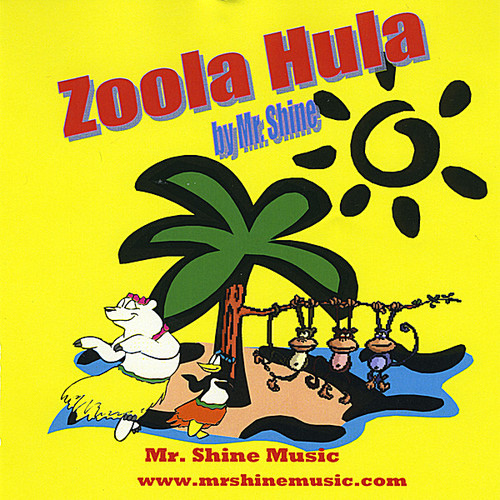The poster for "Zula Hula" features a vibrant yellow background akin to sunshine, with the title "Zula Hula" written diagonally in bold red text with a gray shadow. Directly underneath the title, it reads "by Mr. Shine" in blue text, also shadowed in gray. Positioned just below this text is a black, simplistic sun illustration with radiating rays. Dominating the foreground is a green palm tree situated on a small, cartoon-esque island. Three playful monkeys hang off a long branch extending from the palm tree, their bodies arching towards the water below. To the left of the tree, a polar bear adorned in a grass skirt and a headpiece appears to dance joyfully. Right next to the polar bear, a penguin wearing a blue headband and a grass skirt joins in on the hula dancing. At the bottom of the image, in red text, it reads "Mr. Shine Music" alongside the website "www.mrshinemusic.com". Overall, the graphic resembles an album cover, its playful elements and bright colors suggesting it's designed for children's music.